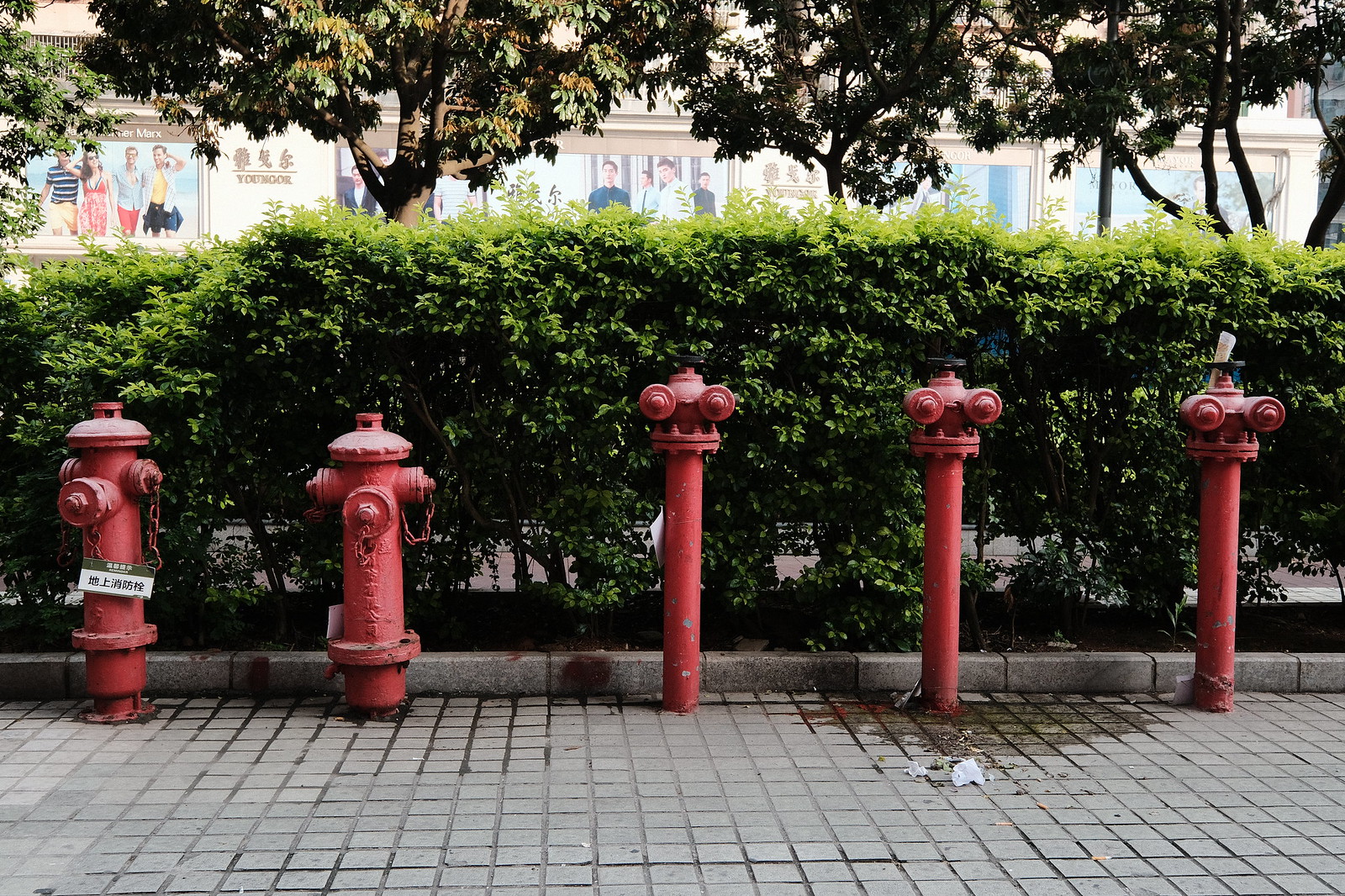This is a color photograph likely taken in an Asian country, featuring five varying red fire hydrants mounted into a gray concrete or tile ground. The first two fire hydrants on the left side are more traditional in appearance, with one of them sporting a tag and a chain. The remaining three hydrants, positioned towards the right, are taller and cylindrical with unique, non-standard tops that diverge from the typical fire hydrant design. Engraved on the fire hydrant furthest to the left is a sign in what seems to be Chinese or Japanese script, which further suggests an Asian locale. 

The backdrop includes green bushes and trees, with a few advertisements visible behind them, likely attached to a building that appears to be a shopping mall. This building features large glass displays with models showcasing outfits. Some of the text on these advertisements is in an Asian language, but there is also an English slogan reading "you more," suggesting the advertising of a store. The overall scene blends elements of urban infrastructure with commercial and natural surroundings.